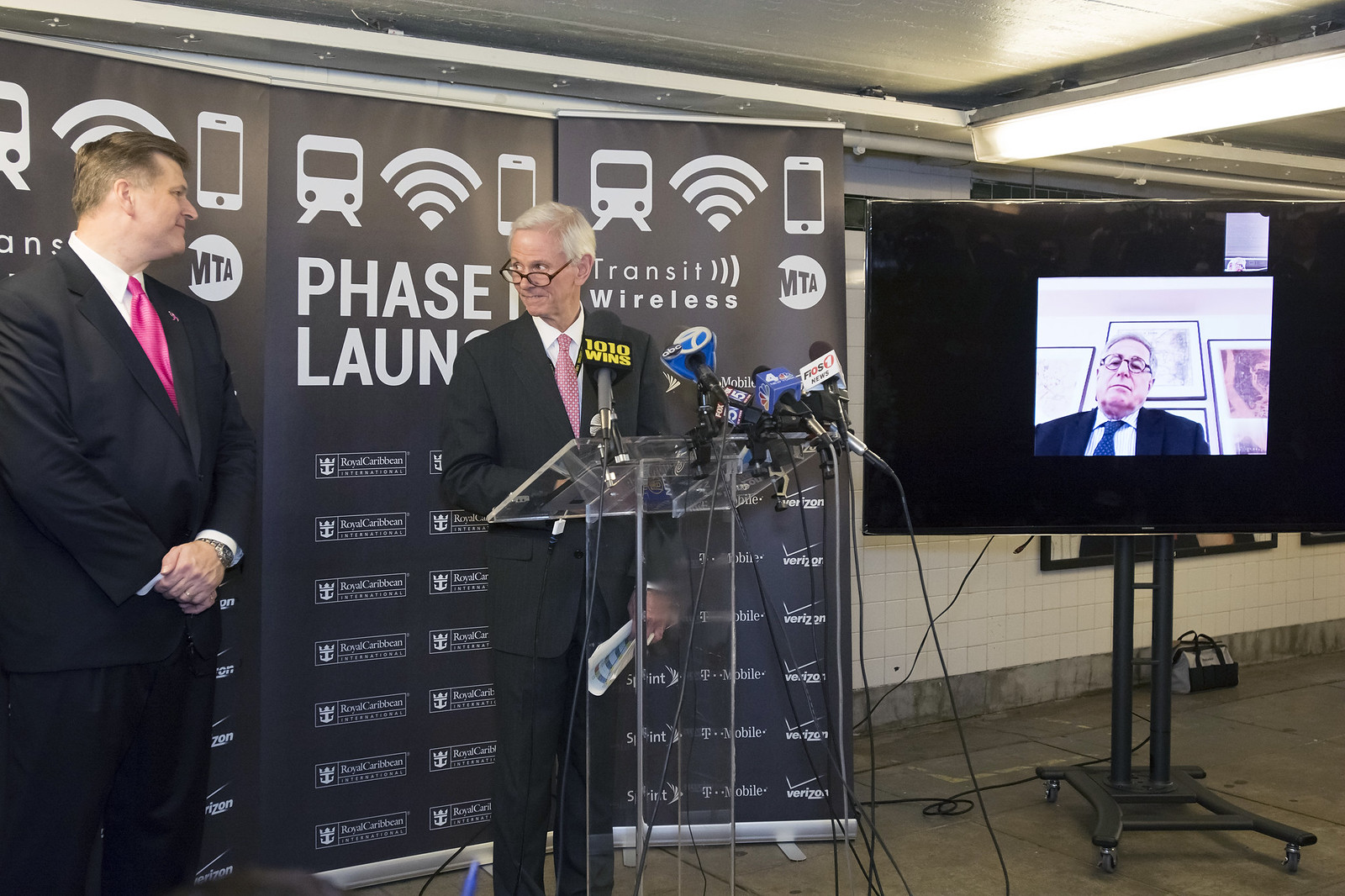The photograph depicts an indoor setting with a stone tile floor and a stone-tiled wall in the background. In the center of the image, an older man stands at a glass podium equipped with about four or five microphones from various media outlets. He wears a gray suit with a light pink tie and is looking off to another man on his left. This second man, dressed in a navy blue suit with a pink tie, is facing the podium. To the right, a man appears on a television screen with a black border, wearing a blue blazer and light blue tie, watching the other two men. The background behind the man on the screen features various plaques and artwork. The scene appears to be during a presentation as indicated by the microphones and the setting, and the colors present in the image include black, white, pink, purple, blue, tan, gray, and yellow. No text is visible, aside from a sign that reads "MTA Phase 1 Launch Transit Wireless," suggesting the context of the gathering. Light fixtures are seen running across the ceiling, indicating the indoor environment.